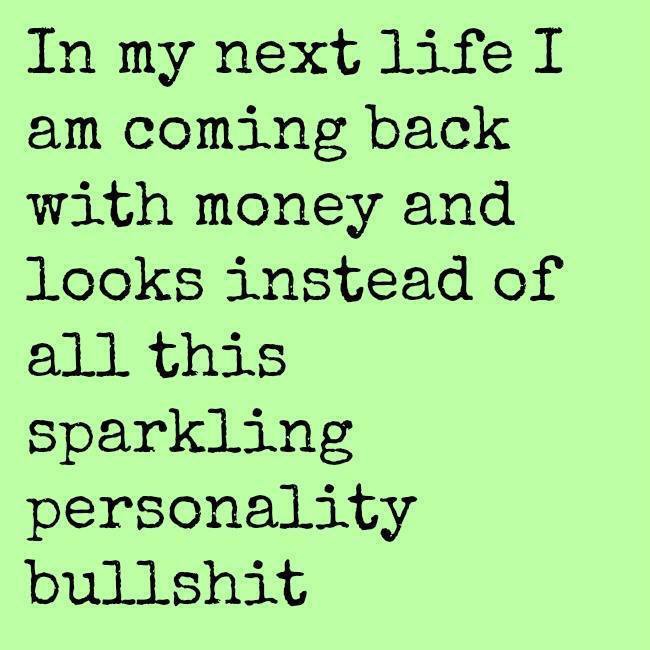The image features a light pastel lime green background, reminiscent of fresh spring grass. Centered on this plain backdrop is a block of black text in simple, typewriter-style font. The text, which is arranged in a nearly perfect square and is straightforward to read, humorously declares: "In my next life, I am coming back with money and looks instead of all this sparkling personality bullshit." The text is large and occupies most of the image. There are no other designs or images, giving the meme a clean and minimalist look. This type of meme is typically seen on social media platforms like Facebook or Twitter, meant to elicit a chuckle with its tongue-in-cheek message.